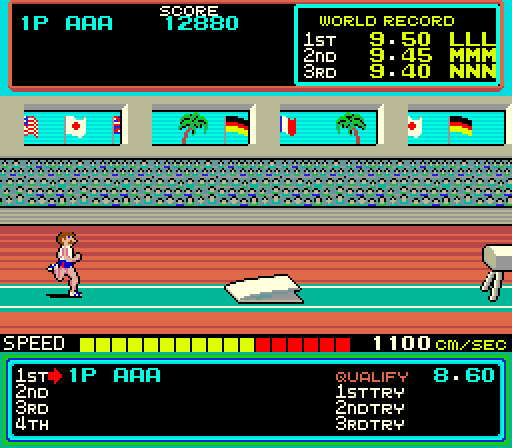The image is a horizontal rectangle showcasing a screen capture from an older-style video game, reminiscent of those from the 80s and 90s, possibly from an Atari or ColecoVision system. The game appears to simulate a gymnastics event, specifically a vault routine. The central focus is a green running track extending from left to right, where a small digital character in a white shirt and blue shorts is running toward a springboard, poised to execute a vault over a white gymnastics horse positioned in the center-right of the frame. Surrounding the track, the indoor stadium's brown floor and gray walls are visible, with an audience implied but not detailed.

In the background, bleachers are adorned with various country flags, including the United States, Germany, Japan, and Italy, interspersed with palm tree graphics. Prominently, a black bar at the bottom of the screen displays rankings and qualifications, reading "1st, 2nd, 3rd, 4th," along with "qualify 8.60." At the top, another black bar provides score information in turquoise and white text, reading "1P AAA" and a score of "12,880." This detailed setup points to a vintage video game screen of a gymnastics or sports competition.